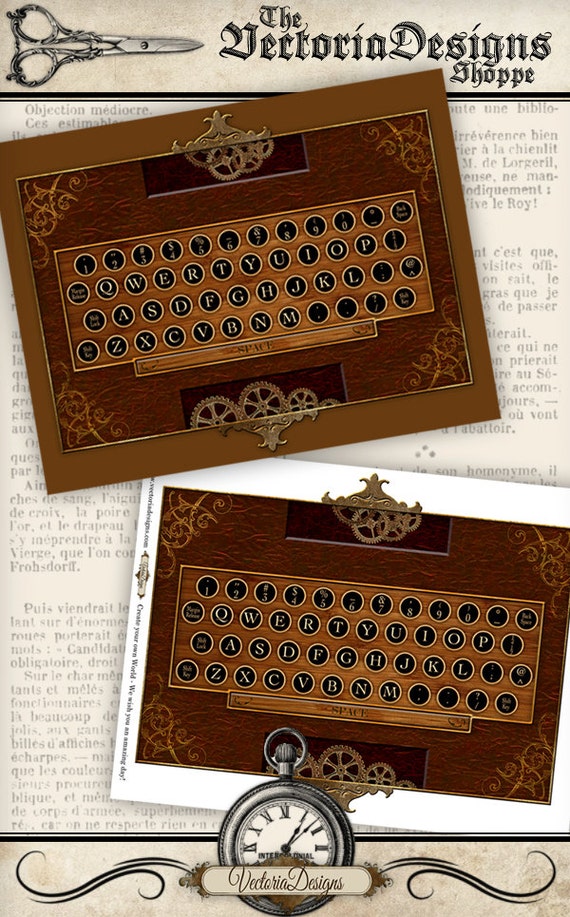The image features a set of vintage typewriter keys meticulously arranged on a brown paper backdrop. These keys, which are possibly for sale or simply displayed for artistic purposes, exhibit a classic design with black backgrounds and white lettering or numbering. Each key is rimmed with metal, adding to their antique charm. 

Framing the entire composition is a triangular frame in a darker brown, embellished with designs in the corners and along the top, resembling intricate gears in a golden hue. This gear-like pattern adds a mechanical and vintage feel to the frame. Surrounding this is another trim also in gold, enhancing the ornate appearance of the image.

At the top center, a pair of silver, old-fashioned scissors with delicate designs can be seen, labeled "The Victoria Design Shoppe" in elegant script. This text is offset to the middle-right side, adding a touch of traditional branding to the image.

Towards the bottom, there is a stopwatch design in silver with black numbers against a white background. Directly underneath, "Victoria Designs" is inscribed in cursive, flanked by swirly motifs on both sides. The bottom section of the paper transitions to a white background, adding visual contrast and balance to the overall composition. 

Filling the middle portion of the image, the beige paper is adorned with black lines near the top and bottom, reminiscent of an old newspaper layout. This background enhances the vintage theme, tying together the elements of typography, antiquity, and craftsmanship.